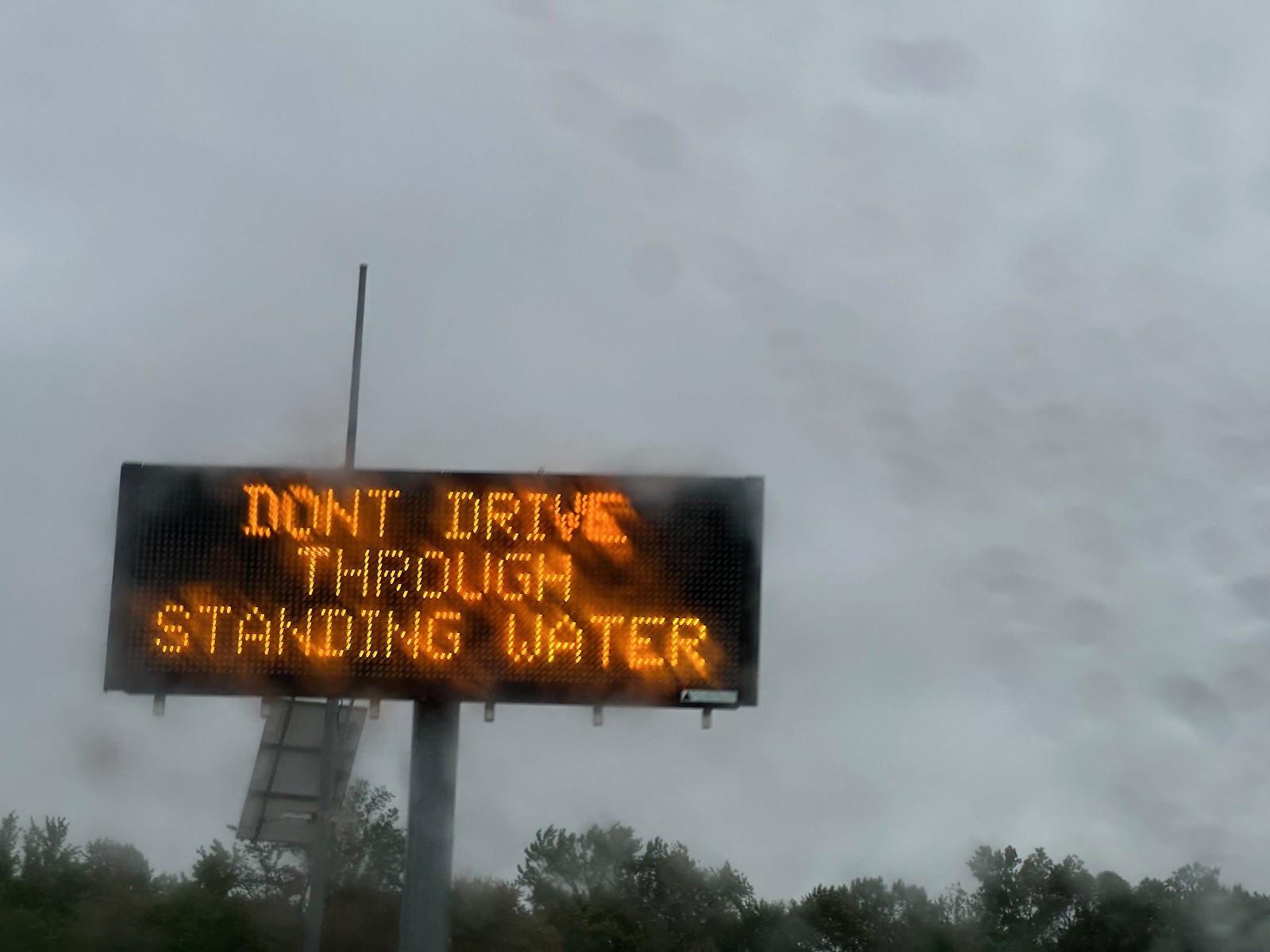A photograph captures a scene through a rain-spattered window, likely from within a vehicle, emphasizing the reflective and watery surface of the glass. The window is dotted with numerous water droplets, adding texture to the image. Beyond the window, a large LED billboard stands tall against a backdrop of a dark, cloudy, and overcast sky. The sign, a black rectangular panel with bright orange lettering, clearly reads, "Don't drive through standing water." The sign itself is high above a barely visible tree line, which forms the horizon with its dark green treetops. Additionally, there are two prominent metal poles and a vertical white sheet connected by metal pipes underneath the billboard, contributing to the structural detail in the scene.